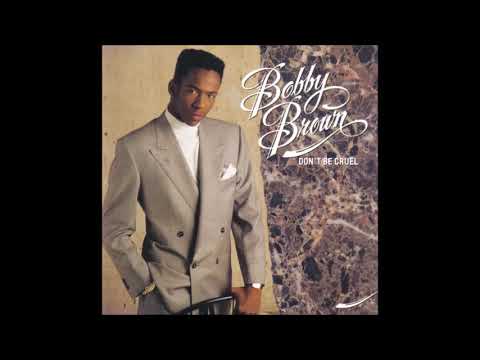The album cover for Bobby Brown's "Don't Be Cruel" features a detailed and striking composition. Bobby Brown is prominently positioned on the left side of the cover, wearing a light gray single-breasted suit paired with a white collared shirt and a white silk pocket square. He sports a flat top hairstyle and has a wristwatch on his left hand. His left hand is resting on a chair, the top of which is faintly visible at the bottom of the image.

The background of the cover is visually split. On the left side behind Bobby is a tan-colored background, while the right features an abstract, marbled pattern with hues of black, light purple, and tan. Bobby Brown's name appears at the top right in a large, elegant cursive font, with "Don't Be Cruel" in a smaller, more conventional font below it, both in white. The entire image is encapsulated by a black border, enhancing the sophisticated presentation of the album cover. The overall aesthetic exudes a classic late-80s vibe, with Bobby Brown confidently looking at the camera, establishing a direct connection with the viewer.